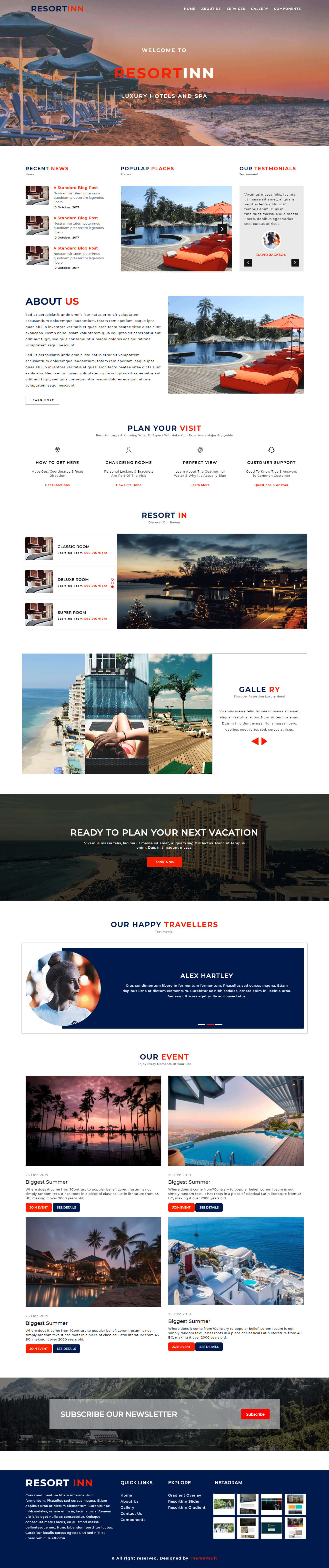**Website Overview of Luxurious Coastal Resort - Result In**

The user interface of the "Result In" luxury hotels and spa website is sleek and inviting. Here is a detailed breakdown of its elements:

**Header and Navigation:**
- At the top left of the page, the phrase "Result In" is prominently displayed, with the word "Result" in blue and "In" in red (styled as "I-N-N").
- The navigation menu features tabs such as Home, About Us, Services, Gallery, and Components.

**Main Image:**
- The main visual is of a serene coastal scene showcasing blue tents and matching chairs stationed on sandy terrain near the ocean. The ocean’s vivid blue color complements the tent setup, creating a harmonious aesthetic.
- Overlaid text reads: "Welcome to Result In, luxury hotels and spa."

**Left Sidebar:**
- The sidebar background is white, featuring a section titled "Recent News."
- Below, it lists "A standard blog post" repeated thrice, all written in yellow.

**Right Sidebar:**
- This area highlights "Popular Places" with a picture of a swimming pool and orange-colored couches and tents.
- It transitions into an "Our Testimonials" section featuring names such as Vimas, Masha, Feliz, and Laknesha. These names appear to be part of a testimonial or review section, written in an unfamiliar language.
  
**Main Content Drilling Down:**
- The "About Us" section includes a descriptive paragraph in a different language, accompanied by a "Learn More" button.
- Another featured image of a blue-hued swimming pool with orange furniture appears here as well.

**Bottom Sections:**
- "Plan Your Visit" area offers practical information and various options: How to Get Here, Changing Rooms, Perfect View, and Customer Support.
- Room categories listed include Classic Room, Deluxe Room, and Super Room.
- A "Gallery" section prompts visitors with "Ready to plan your next vacation?" followed by a "Patronage Now" button.

**Customer and Event Segments:**
- "Our Happy Travellers" emphasizes testimonials from guests like Alex Headley.
- "Our Event" section highlights upcoming events, each featuring "Join Event" (red button) and "See Details" (blue button). There’s a notable event titled "Biggest Summer" dated 25th December 2019.

**Footer Details:**
- A "Subscribe to our newsletter" call-to-action includes a red "Subscribe" button.
- The footer reiterates "Result In" with more descriptions in a different language.
- Additional navigation links provided include Quick Links, Explore, Instagram, Home, About Us, Gallery, Contact Us, Component, Gradient Overlay, Result In Slider, and Result In Gradient.

This detailed layout paints a comprehensive picture of what visitors can expect from their experience at "Result In," encapsulating the essence of luxury and attention to detail.